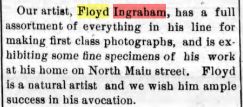This is a tiny rectangular excerpt from a newspaper, displaying a scanned portion against a grayish-white background. The image is bordered on both the left and right sides by thin, black vertical lines. The black, bolded paragraph inside starts with an indent and reads: "Our artist, Floyd Ingraham, has a full assortment of everything in his line for making first-class photographs, and is exhibiting some fine specimens of his work at his home on North Main Street. Floyd is a natural artist, and we wish him ample success in his avocation." The name "Floyd" at the beginning is highlighted in yellow, while "Ingraham" is highlighted in pale red.